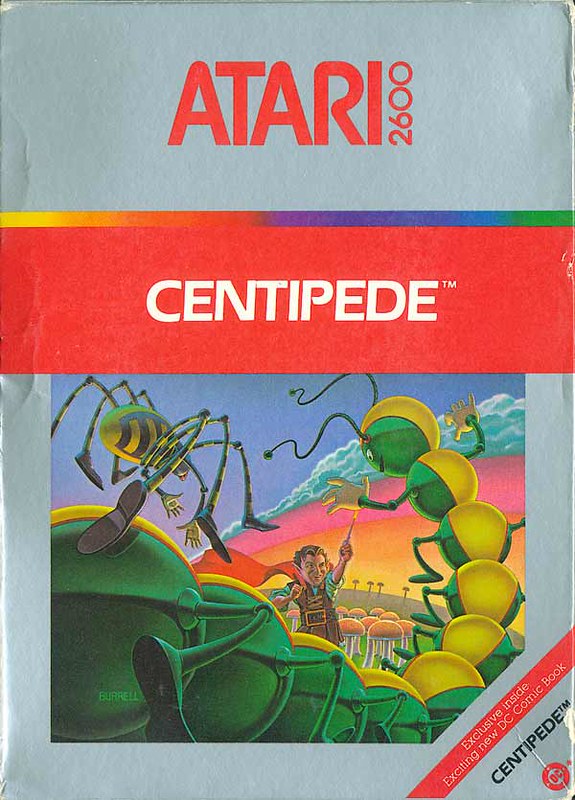This is a video game box for the classic Atari game "Centipede." The top portion of the box features a horizontal gray block displaying the word "Atari" in bold red letters. Below this, the vertical text "2600" runs along the "I" in Atari. A vibrant rainbow stripe lies beneath the gray block, followed by a thick red stripe with "Centipede" written in white letters, along with "TM" positioned in the upper right of the word.

The main image below this header showcases a detailed, cartoonish scene: a long, segmented centipede and an additional insect resembling a spider. A wizard-like figure in a brown tunic with lace detailing, a black belt with a gold buckle, and a flowing red cape is depicted pointing a wand at the centipede. This figure stands among numerous mushrooms with green grass visible at their bases. The artwork is bordered by a gray frame.

In the lower right section of the box, a red and white band highlights the text "Exclusive inside, exciting new DC comic book," with the word "Centipede" and "TM" in black letters within a gray triangle below it. Adjacent to this text is a circular DC logo, featuring "DC" in red letters on a gray background. The circle is outlined in red with white dots at its compass points, angled at 45 degrees to the upper left. Just outside the DC circle is a red blotch positioned to the right.